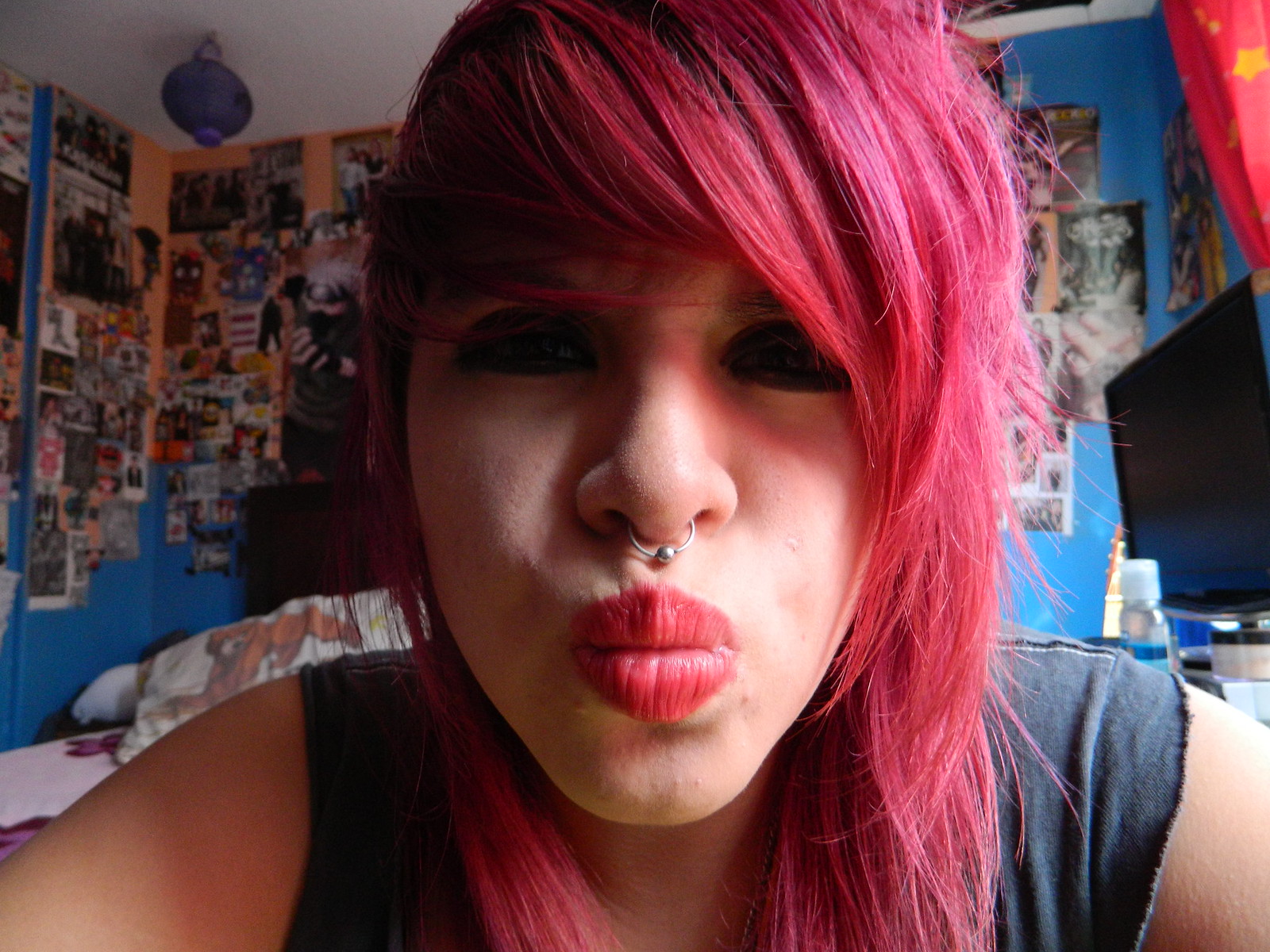The image is a detailed, realistic photograph of a young Caucasian woman taking a selfie in her bedroom. She is the primary focus of the picture. The woman has shoulder-length, pink hair combed forward over her bangs, which partially obscure her eyes enhanced with dark black eyeliner. Her other prominent facial features include a nose ring with a small metal bead that sits in the septum, and she’s wearing red lipstick that closely matches her hair color. She is dressed in a black, sleeveless tank top and is making a kissy face towards the camera.

The backdrop of the image is a blue-walled room adorned with several posters and photos, which are hard to discern in detail. There is also a flat-screen TV situated in the bottom right corner of the image. The left side shows part of a bed with white sheets and pillowcases, and toward the right side, the illumination suggests the presence of a window, partially covered by red curtains with yellow stars. The photo captures the intimate and personalized space of the bedroom, filled with hints of the woman’s personality and style.